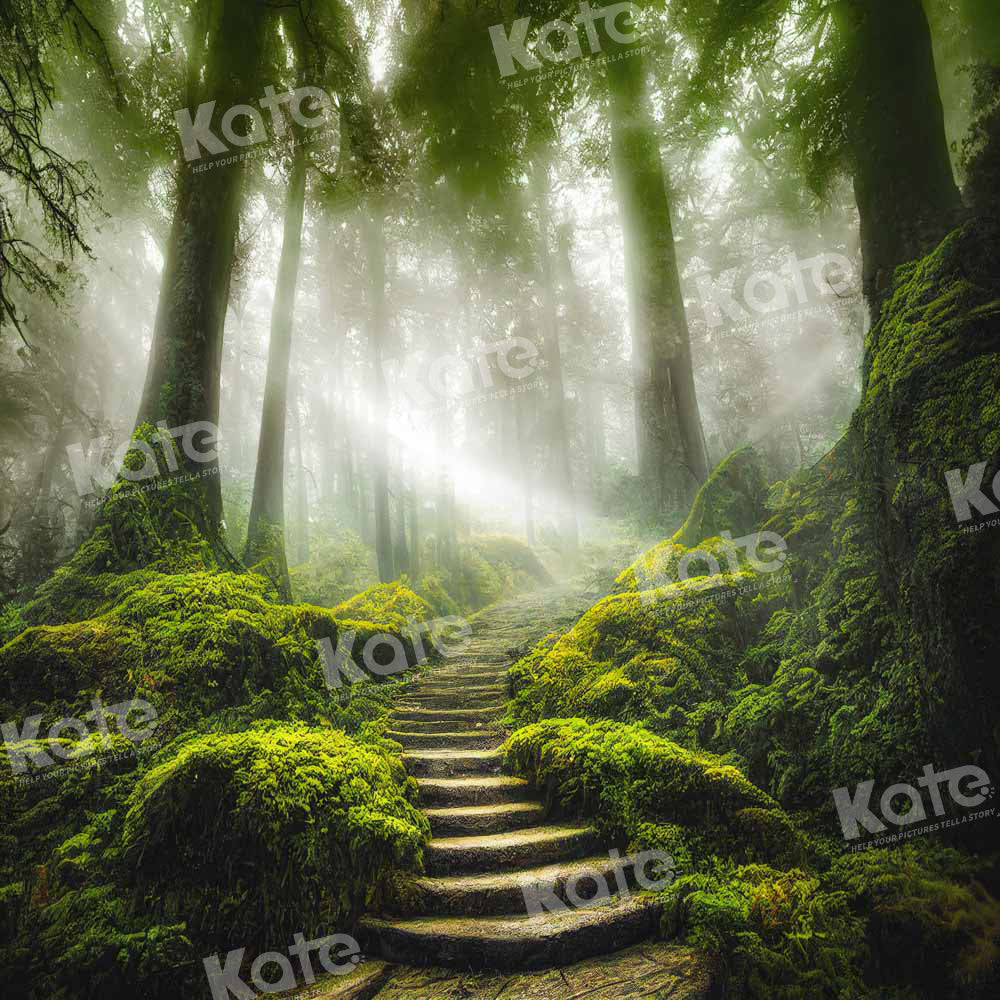A stunning and ethereal photograph captures a dense, mossy forest. Centrally placed in the image is a stone staircase that starts from the foreground and curves slightly to the right as it ascends. On either side of the stone steps, lush greenery and moss-covered boulders encroach upon the path, their leafy and fuzzy textures contributing to the forest's mystique. The stone steps are bathed in dappled sunlight, which filters through the thick canopy of tall, thin trees. This interplay of light highlights sections of the moss and stairs in a yellowish-green hue. The background is filled with towering trees whose leaves form a vast canopy, allowing streaks of sunlight to create a misty, almost smoky atmosphere. The lower part of the image remains in shadow, further emphasizing the magical light shimmering through the upper half. The photograph is adorned with multiple instances of a watermark that reads "CATE" in large letters, with some smaller, less distinguishable wording beneath, indicating the photographer's signature.